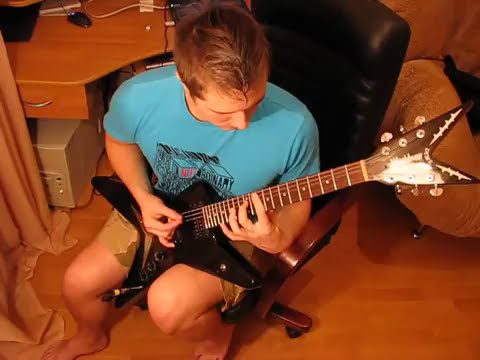The photograph captures a man, possibly a young adult, playing an electric guitar in what seems to be a dorm room or a bedroom. The image is taken from an elevated vantage point, perhaps from a bunk bed, showing the top of his head and a detailed view of his surroundings. The man, who has light brown, almost blond hair styled into a slight mohawk, is barefoot and dressed in khaki-colored shorts and a turquoise blue, short-sleeved shirt with a black artistic design that includes unreadable letters. He is seated on a black rolling office chair with wooden armrests. His left hand forms a chord on the dark brown neck of the guitar, while his right hand picks at the black, angular, star-shaped body of the instrument. The room features a wooden floor, a light brown desk with a computer tower beneath it, a black mouse with a cord on the desktop, and to the right of the chair, a tan, plush beanbag chair. Scattered on the floor, there appears to be a curtain or towel. The overall setting, with its casual and lived-in vibe, strongly suggests a dorm room environment.